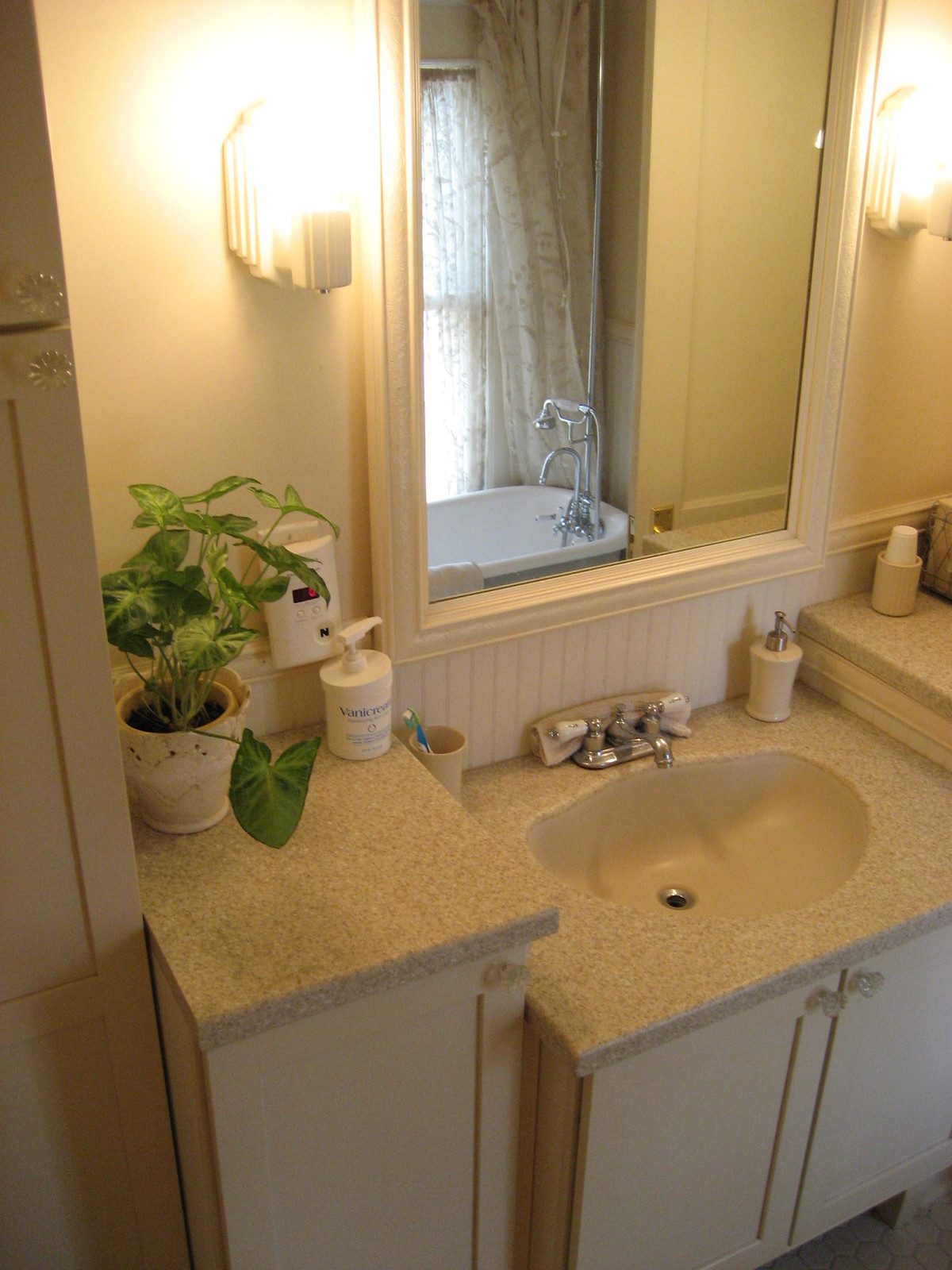The image captures an intricately detailed view of a bathroom, with the camera positioned slightly from the left corner and angled down and to the right. Dominating the foreground on the left side is a cabinet. The upper cabinet is partially visible, featuring a clear handle on the bottom right. Below it, the lower cabinet is shown more fully, extending from about a third of the frame's top to the bottom, adorned with a gold handle.

To the right of the cabinet is a white wall. Approximately an inch from the top edge of this wall, a white light fixture extends towards the camera, casting a warm glow. Adjacent to the light fixture is a mirror surrounded by a white border, reaching down to the sink’s baseboard. The mirrored reflection reveals a portion of a bathtub in the bottom left corner, with the bathtub faucet centered in the mirror. Above the faucet, there is a glimpse of a window with light streaming through a curtain.

Below the mirror is a marble sink, featuring a silver faucet flanked by white handles. To the left of the faucet is a cup holding a toothbrush, while to the right sits a brown soap dispenser with a silver top. Continuing to the right, a small ledge showcases a brown cup with a white cap. On the left side of the sink, another marble counter hosts a white pot with a lush green plant, and something is plugged into the wall nearby. Below and slightly to the right, a small white bottle with a squeeze top is positioned.

Finally, the front of the sink area is notable for two doors that open outward from the center, with a large door on the cabinet featuring a handle in the top right corner.